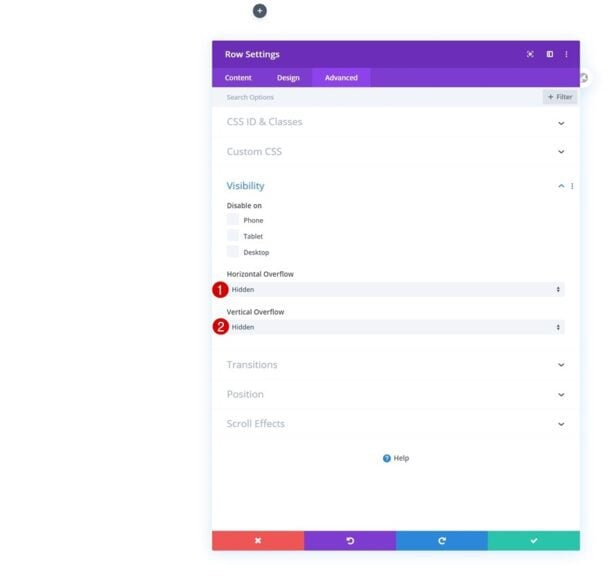Screenshot Description: Advanced Row Settings Panel in a Web Design Interface

The screenshot depicts the "Advanced Row Settings" panel of a web design interface, presented in a structured layout with multiple sections and options. 

At the top of the panel, there is a prominent navy blue circle featuring a plus sign in its center, likely representing an add or expand function. Below this, in a purple bar, is the label "Row Settings" written twice, stacked one above the other. To the right of this label, three small icons are visible: the first is a box with a dot inside, the second appears as a square, and the third comprises three vertical dots, although the icons are somewhat blurred and hard to distinguish clearly.

Beneath the purple bar, there are three clickable tabs aligned horizontally, also in a purple bar: "Content," "Design," and "Advanced." The "Advanced" tab is currently selected, which brings its contents into focus. Below these tabs, there is a light gray box labeled "Search Options," with a darker gray square on its right containing a plus sign and a filter icon.

The main section of the interface includes several categories with dropdown menus and options:
1. **CSS ID and Classes**: Includes a dropdown on the right.
2. **Custom CSS**: Features a dropdown on the right.
3. **Visibility**: Highlighted in blue with a dropdown expanded upwards, displaying options to disable visibility on various devices. Under this, there are checkboxes for "Phone," "Tablet," and "Desktop," none of which are selected.
4. **Horizontal Overflow**: To the left of this item, there is a red circle with a number 1, and to the right, the option "Hidden" is shown with up-and-down selection triangles for choosing other settings.
5. **Vertical Overflow**: Similar to horizontal overflow, this item has a red circle with number 2 on the left and the option "Hidden" with selection triangles on the right.

Following these are sections labeled "Transitions," "Position," and "Scroll Effects," each accompanied by dropdown menus.

At the bottom of the panel, there is a blue circle with a question mark inside it, labeled "Help," to provide users guidance. Below this, there are four colored action bars: 
1. A red bar with an X, representing cancel or delete action.
2. A purple bar with a circular arrow pointing left, indicating a backward navigation function.
3. A blue bar with a circular arrow pointing right, signifying forward navigation.
4. A mint-colored bar with a checkmark, likely used to confirm or save changes.

The overall interface is robust, providing extensive settings and customization options for users to manage the advanced settings of their web design elements.